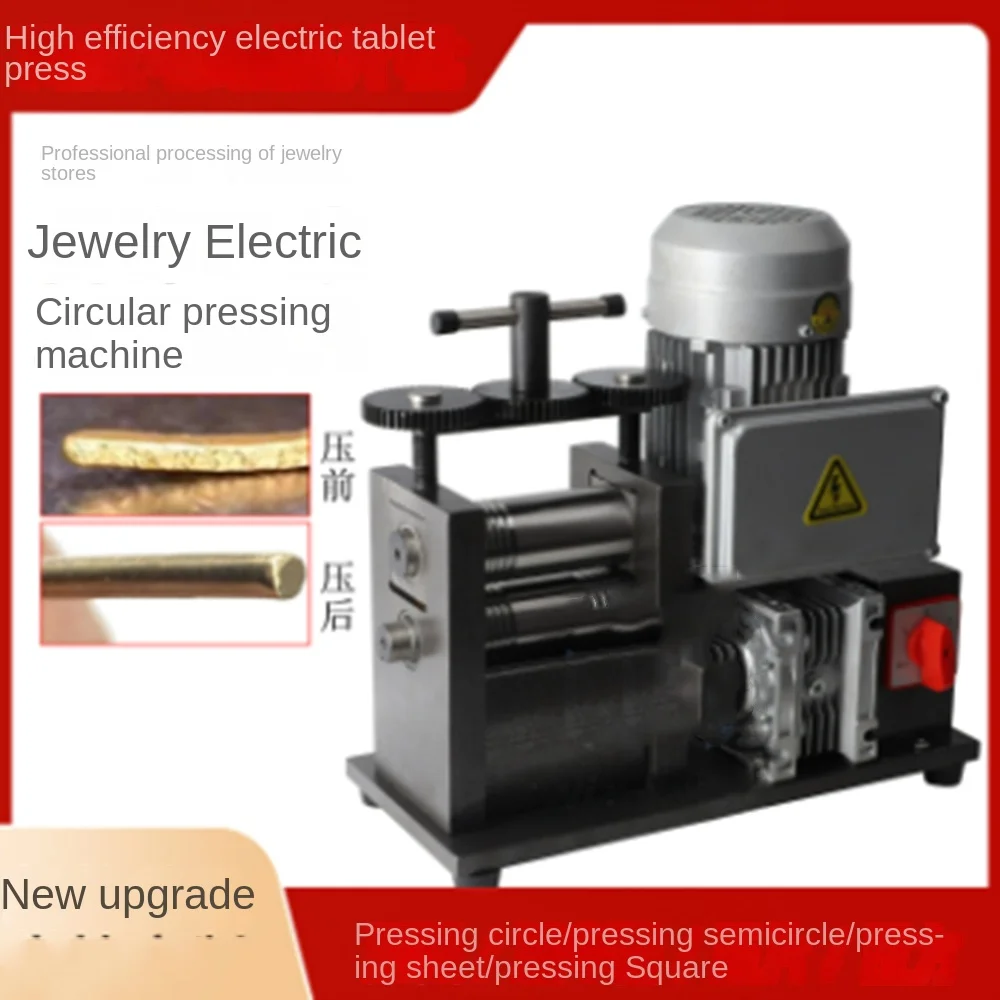This advertisement features a high-efficiency electric tablet press, prominently displayed against a sleek, indoor backdrop. The text in the upper-left corner reads "High Efficiency Electric Tablet Press" in bold white letters on a red background. Below it, in smaller, dark letters, the text declares "Professional Processing of Jewelry Stores," followed by "Jewelry Electric Circular Pressing Machine" in large black letters. 

The central image is a detailed photograph of the machine itself, a state-of-the-art silver device perched on a black platform with four small legs. At its top, a handle is connected to a series of three flywheels, designed to operate the press mechanism. On the right side of the machine, a red button serves as the on/off switch next to gray, plastic components, including clamps and bellows. 

The machine includes a tray adorned with a safety symbol, indicating its secure operation. The text along the bottom of the image emphasizes its versatile pressing capabilities: "Pressing Circle / Pressing Semicircle / Pressing Sheet / Pressing Square," with "New Upgrade" highlighted in the bottom-left corner. 

Supplementary images depict a transition from a flat piece of metal to a transformed spherical gold object, illustrating the machine's functional prowess. Although some oriental characters are present on the images, their meanings are not immediately clear.

This comprehensive image and text combination underscores the high-efficiency electric tablet press's suitability for precision jewelry processing while offering multiple pressing options for diverse applications.